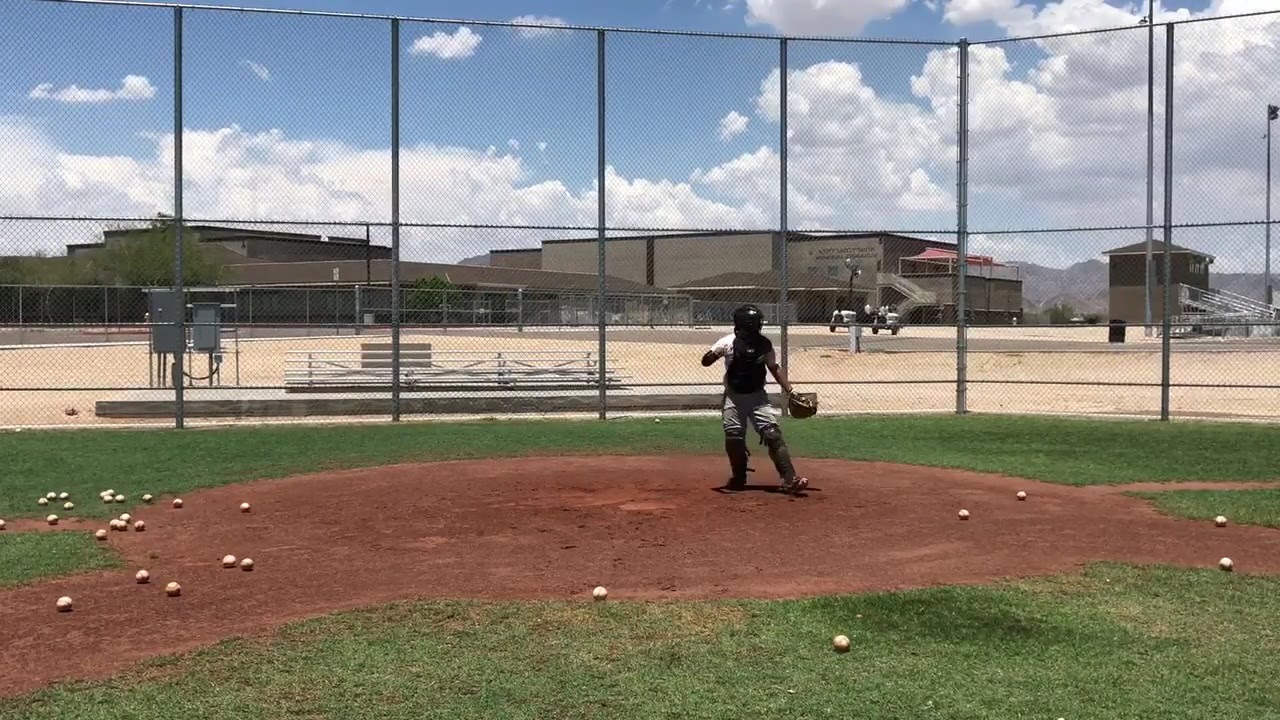In this daytime photograph, we see a catcher positioned on a baseball field. The ground consists of short green grass with a prominent circular dirt patch extending to the left and right, particularly filled with numerous baseballs, mostly on the left-hand side but also scattered on the right and lower end of the image. The catcher stands out in the center, clad in a typical baseball uniform complete with knee pads, a chest pad, and a face mask, and they're holding a catcher's mitt in their left hand. The catcher is somewhat shadowed, giving a sense of the sun being high above. Behind the catcher is a two-story high chain-link fence with stands and industrial-looking buildings beyond it. The background showcases a dirt field, a few hills or mountains hinting at a possible desert environment, all under a broad blue sky dotted with thick white clouds.